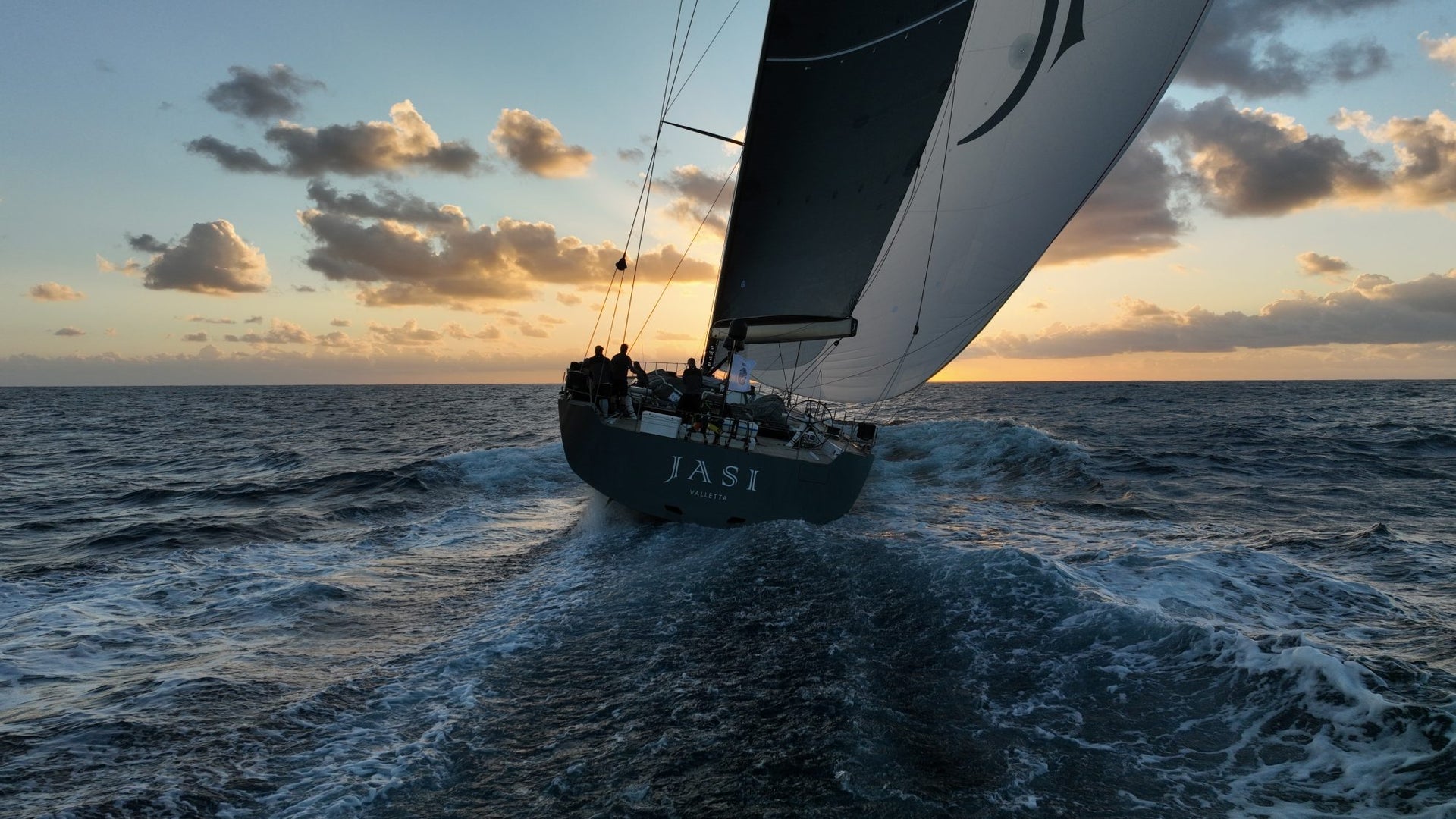The photograph captures a dynamic scene of a sailboat navigating through a stormy sea. The boat, viewed from the aft, bears the name "J.A.S.I." prominently on its blue-painted stern. Several crewmen are visible as small black silhouettes moving around on the deck. The vessel features a striking sail configuration: a large white sail on the right adorned with a curved line pattern and a smaller black triangular sail. The sail extends upward, though its top is cut off by the frame of the photo. The surrounding sea is turbulent, with waves and foam adding to the sense of motion. The sky above is a dramatic mix of blue with patches of white and grey clouds, illuminated by golden light suggestive of either sunrise or sunset. The horizon cuts the image almost symmetrically, dividing the choppy waters below from the swirling atmospheric drama above.